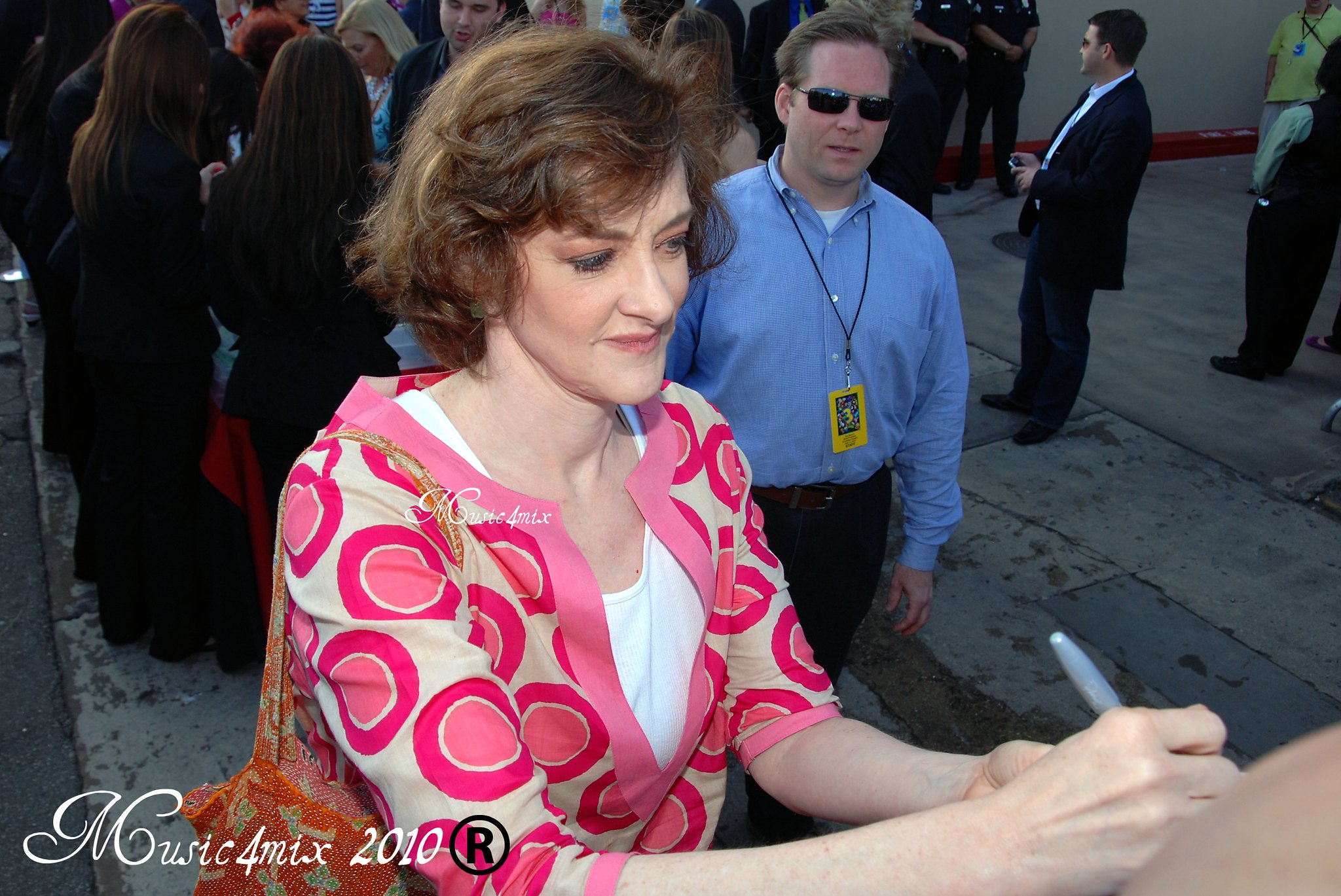In this vibrant outdoor scene set in the middle of the day, a middle-aged, skinny woman with medium-length, slightly wind-tousled brown hair is prominently featured in the center. She is dressed in a multicolored, thin jacket over a white blouse, with an orange bag slung over her shoulder. The woman, possibly an actress, is signing something with a marker in her right hand, possibly a piece of skin or a poster. She has makeup on and features such as a big nose are visible. Beside her, to the right, stands a larger man who appears to be a bodyguard, wearing sunglasses, a blue shirt, dark pants, and a lanyard with a badge that displays the number "three." Surrounding them is a large crowd of people, some dressed in suits and holding their phones, presumably to capture the moment. The ground beneath them consists of stone tiles. At the bottom left of the image, the text "music for Mix 2010" is visible, along with a circle containing an "R." The image is awash with a palette of various colors, including shades of pink, white, black, light blue, yellow, green, and gray.